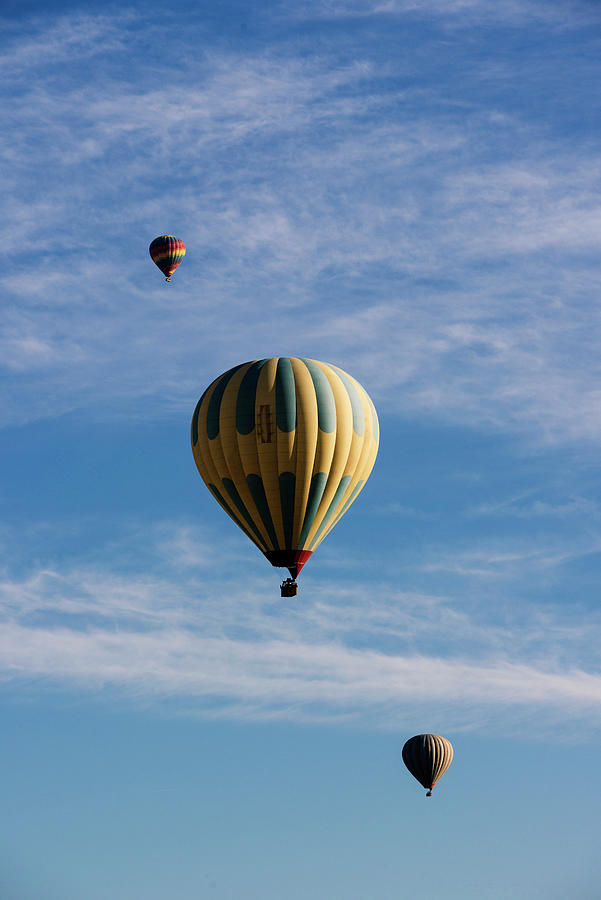In a bright blue sky adorned with light, wispy white clouds, three hot air balloons are in flight. Dominating the center of the image is a large yellow balloon with blue stripes on its top and bottom, divided by a yellow section in the middle. The balloon's basket, silhouetted against the balloon, adds to the scene. To the upper left, a smaller balloon with vertical blue, yellow, and orange stripes hovers in the distance, while in the lower right, another distant balloon, brown with white stripes, floats against the serene sky. The translucent clouds provide a gentle, airy backdrop to the vibrant colors of the balloons.